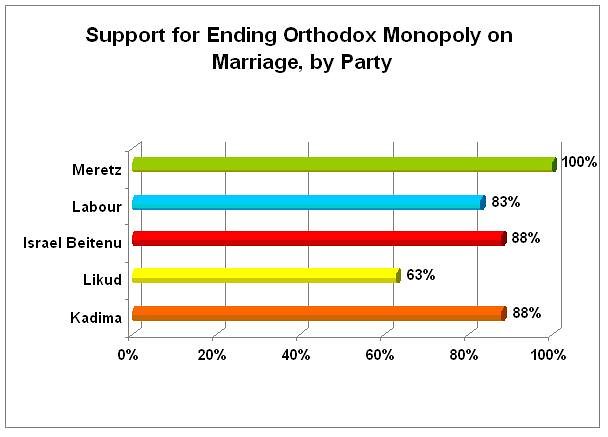The image is a white card bordered in black that features a detailed graph with the title "Support for Ending Orthodox Monopoly on Marriage by Party" at the top. The graph illustrates support levels for various political parties, marked by colorful horizontal lines. On the left side, the parties listed are Meretz, Labor, Israel Beitenu, Likud, and Kadima. Meretz is represented by a green line reaching 100%, Labor by a blue line at 83%, Israel Beitenu by a red line at 88%, Likud by a yellow line at 63%, and Kadima by an orange line also at 88%. The horizontal axis at the bottom of the graph displays percentage intervals from 0% to 100% in increments of 20%. The combination of vibrant colors and distinct percentages visually communicates the varying levels of support each party has for ending the Orthodox monopoly on marriage.